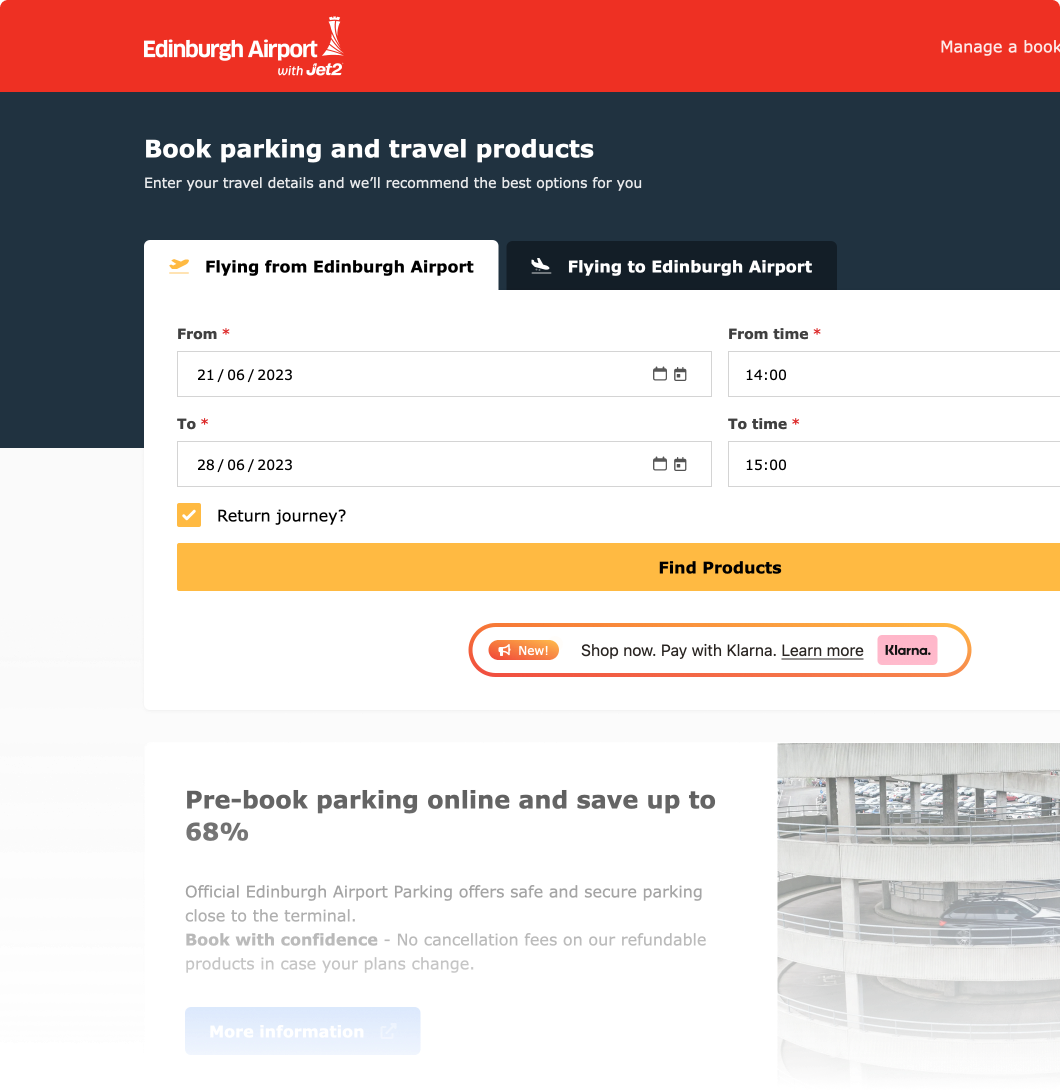The image depicts a partially cropped booking form for travel services associated with Edinburgh Airport, created by Jet2. The form is visually divided into several sections:

1. **Header**:
   - A horizontal red stripe spans from the upper left to the upper right, emblazoned with the text "Edinburgh Airport with Jet2."
   - In the upper right corner, the text "Manage a booking" appears, though it is partially cut off in the image.

2. **Body**:
   - The next section features a black background and includes instructions: "Book parking and travel products. Enter your travel details and we'll recommend the best options for you."
   - There are two tabs for selecting flight details:
     - The left tab, highlighted in white with bold black text, reads "Flying from Edinburgh Airport."
     - The right tab, in black with white text, reads "Flying to Edinburgh Airport." The active tab is the one on the left.

3. **Booking Details**:
   - A form for entering travel dates is provided:
     - Departure Date: 21/06/2023, Time: 14:00
     - Return Date: 28/06/2023, Time: 15:00
   - An orange checked box is labeled "Return journey," indicating that this is a two-way ticket.

4. **Action Button**:
   - There is a prominent button labeled "Find products." Despite its large size, the text is in small font, causing it to appear disproportionate.

5. **Promotional Section**:
   - Below the button, a promotional message reads: "New! Shop now, pay with Klarna."
   - Another promotional note suggests pre-booking parking online to save up to 68%.

Overall, the image is an interface for booking flights and associated services, highlighting various options and promotional offers for travelers using Edinburgh Airport.